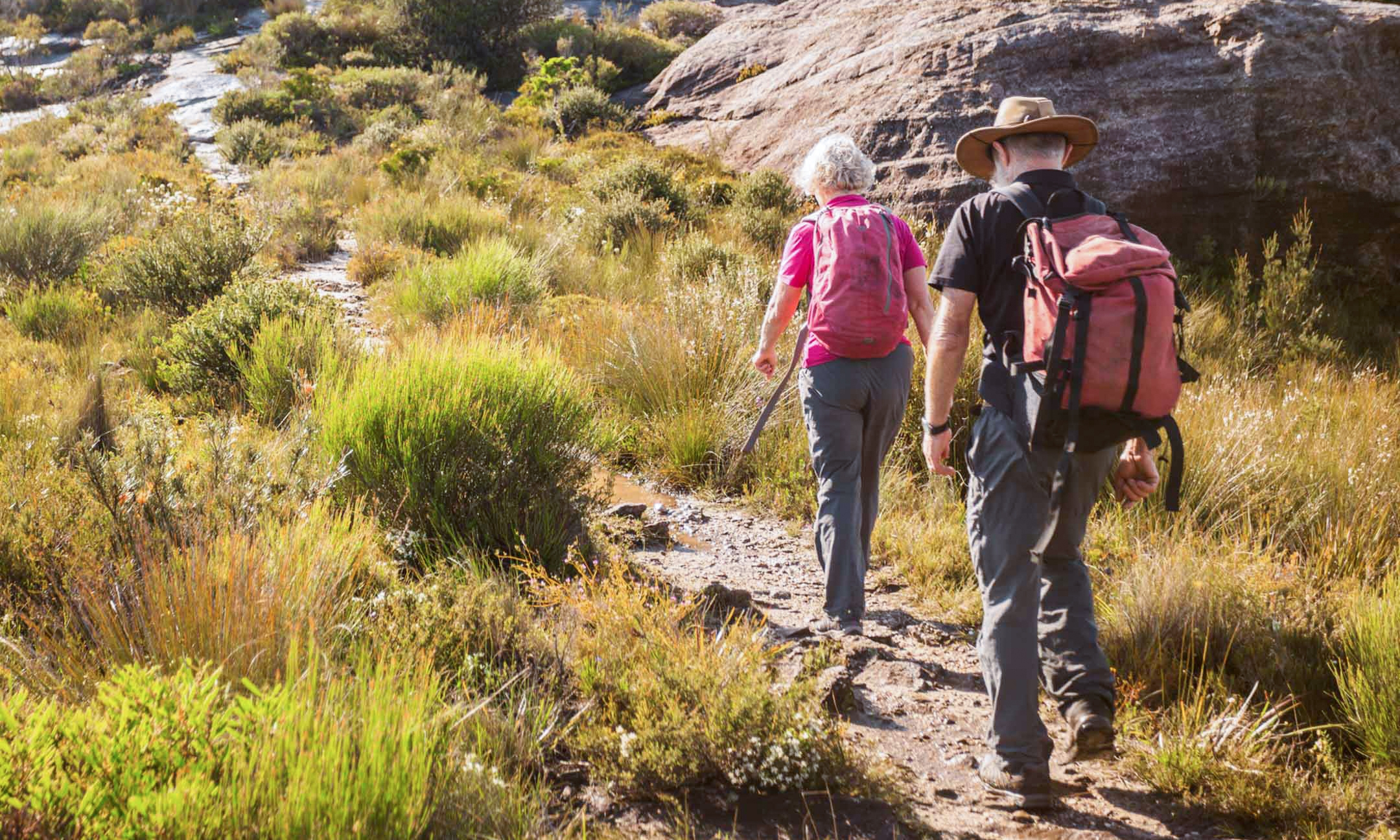The photograph captures an older couple hiking up a rocky, dirt trail surrounded by a mix of yellow, green, and brown shrubs and grasses. The trail, which features patches of brown-colored water, winds up a slope that extends from the rocky path in the top left corner of the image to the bottom right. The woman, who leads the way, has short white hair and wears a pink short-sleeved t-shirt along with gray pants. She carries a pink backpack. Behind her is the man, wearing a black t-shirt, gray pants, brown boots, and a tan sun hat. He has a coral-colored backpack. Both are looking down at the ground as they walk. To the right of the trail, there is a large gray boulder with more sparse weeds growing around it. This scene showcases their journey through a serene and rugged landscape.